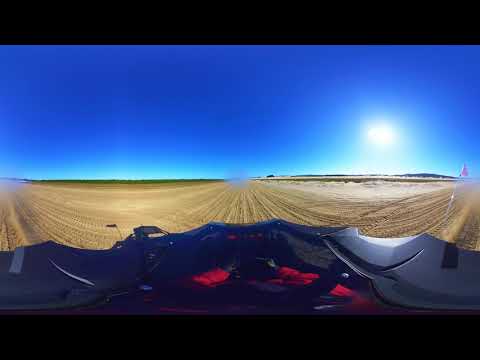The image, taken from a first-person perspective, captures someone driving what appears to be an off-road vehicle like an ATV or dune buggy. The black handlebars of the vehicle are held by a person wearing a vibrant red jacket and black gloves. The scene is bathed in the bright light of a clear, cloudless sky, with the sun prominently shining on the right side of the image. The terrain is flat and expansive, resembling farmland or prairie, characterized by dark, sandy soil and numerous straight tire tracks crisscrossing the dirt road. In the middle and far distance, there is an endless expanse of green fields, suggesting farming fields or grasslands. The horizon also shows a thin sliver of grassy area on the left and more dirt to the right. Notably, the image has thick black borders at the top and bottom, framing the panoramic view. The sky features a gradient from a deep blue at the top to a lighter blue near the horizon. The overall impression is one of solitude and vast open space under a stunning blue sky.